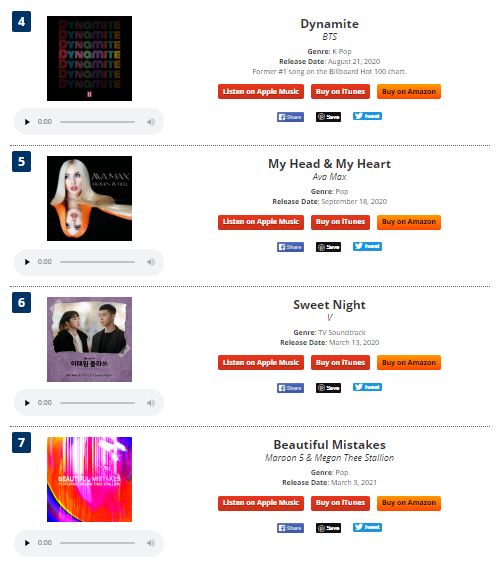This is a detailed screenshot showcasing a selection of songs on a music website. 

In the top left-hand corner, there's a dark navy blue box featuring a white forward arrow symbol. Adjacent to it is an album cover titled "Dyno Might" displayed in vibrant rainbow colors. The text "Dyno Might" appears in the middle with a mirrored gradient effect that gets darker from top to bottom. Below the album cover, there is a gray oval containing a black play button labeled "0:00," a progress bar displaying the length of the song, and a speaker icon. The text "Dyno Might" is printed in bold black on the left side of the album cover’s central section, followed by "BTS" and "John Rae" also in bold. Additionally, it notes that "Dyno Might" is a K-Pop genre song released on August 21, 2020, and was a former number one on the Billboard Hot 100 chart. There are action buttons in red for "Listen on Apple Music," "Buy on iTunes," and an orange button for "Buy on Amazon." Social media share buttons are also present: Facebook, Twitter, and an unidentified middle black button.

Following is another album cover for "Ma Max" against a navy blue background with a white "5." The cover features a woman's head with blonde hair on the top half and a mirrored image of a woman's head with red hair on the bottom half. Below this cover is a play button labeled "0:00" with a progress bar and a speaker icon. The song title is "Born," by Ava Max, within the pop genre, released on September 18, 2020. Similar action and sharing buttons follow, with "Listen on Apple Music," "Buy on iTunes," "Buy on Amazon," Facebook, and a Tweet button.

Next in the sequence is another navy blue box with white text labeled "Sweet Night." The album cover is predominantly purple and depicts a man and a woman standing and slightly facing each other. Below this cover is a play button, and in bold, the text "Sweet Night" and then "B." The song falls under the TV soundtrack genre and was released on March 13, 2020. The action buttons for this song include "Listen on Apple Music," "Buy on iTunes," "Buy on Amazon," and sharing options through Facebook, a black share button, and Twitter.

Lastly, there is an album titled "Beautiful Mistakes," featuring mostly orange and red tones in a design that resembles the side of a ball with white light shining through glass, and some blue in the upper right and bottom left-hand corners. The song "Beautiful Mistakes" is by Maroon 5 and Megan Thee Stallion, categorized under the pop genre and released on March 3, 2021. Action and sharing options follow similarly, with "Listen on Apple Music," "Buy on iTunes," "Buy on Amazon," and share options through Facebook, a black share button, and Twitter.